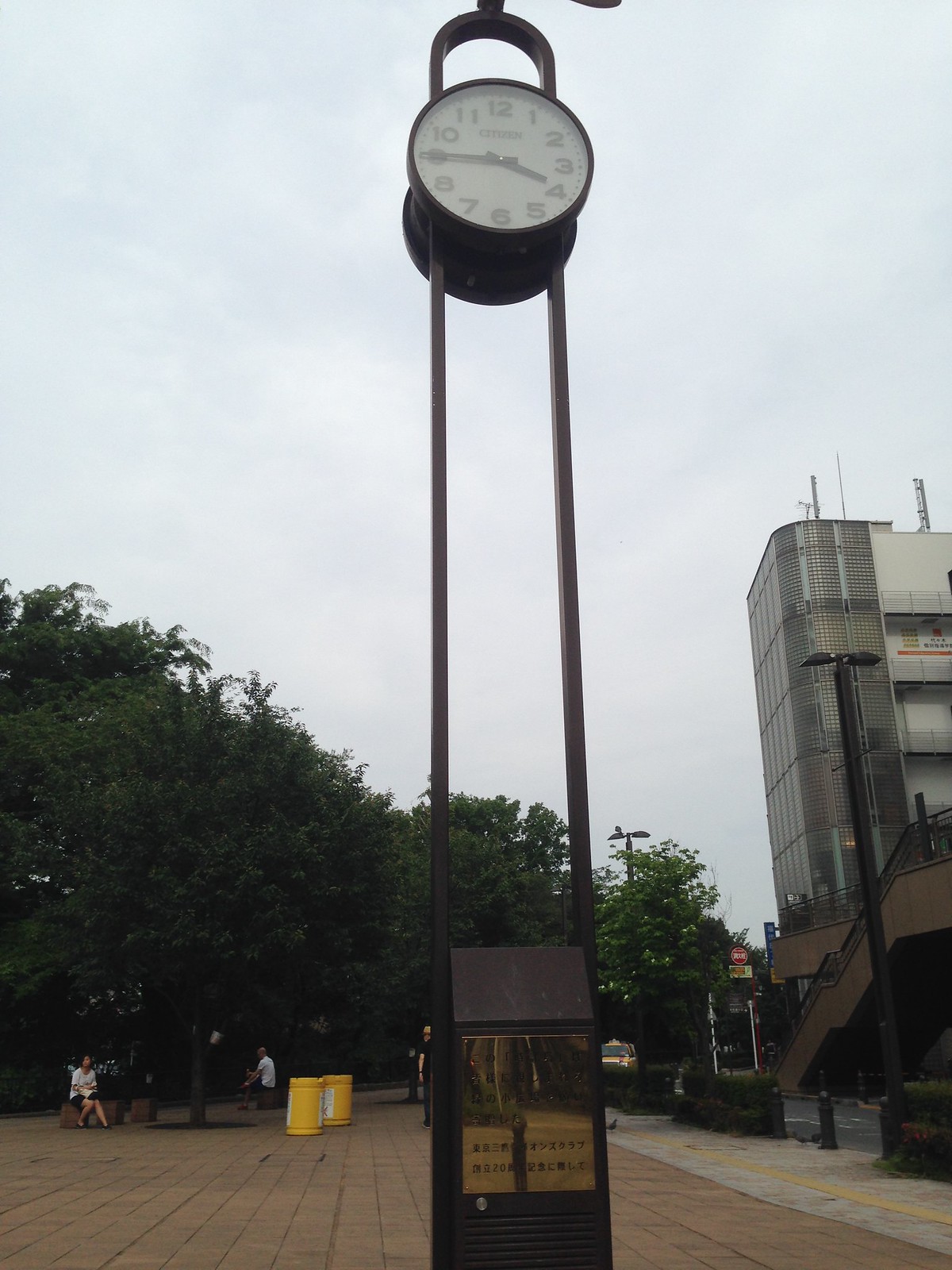This color photograph captures a tall outdoor clock situated in an open courtyard bustling with people. The clock is supported by a brown, sturdy structure with a thick, weighted base. Two metal poles rise from the base, supporting the clock, which has a round, white face with black numbers and hands indicating the time is a quarter to four. The sides of the metal structure loop at the top, but the image is cropped at this point. There's an inscription on the clock face, but it's not legible. The courtyard features terra cotta-colored tile pavers laid closely together, creating a cohesive ground surface. In the background, there are two yellow garbage cans adorned with posters that cannot be clearly read. Various people animate the scene; a woman is seated on a bench, seemingly alone, while a man near the clock structure appears to be throwing something at its base. A copper-colored metal placard, which is square in shape, is affixed to the base of the clock structure, but its text is not readable in this image.